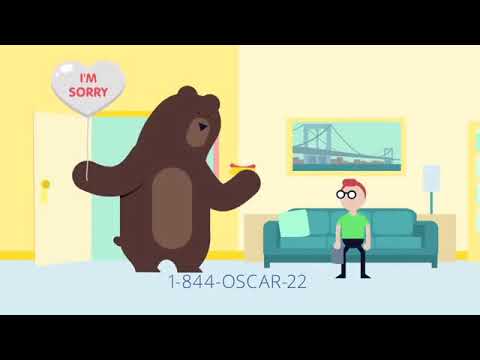In this cartoon-style graphic art, a tall brown bear with a lighter brown muzzle and belly stands on the left, holding a heart-shaped balloon in its right paw that says "I'm sorry." The bear's left paw is raised. Behind the bear is an open beige door, through which a blue background can be seen. On the right side of the image, a man with red hair, wearing black-framed glasses, a lime green short-sleeved t-shirt, and black pants, sits on a green couch. The couch has a green pillow, and there's a coffee table with a lamp with a white shade beside it. Behind the man, the wall is beige, adorned with a picture of a beach. On the left side, the wall is yellow. A gray floor and a low-detailed, cartoonish style tie the scene together. At the bottom of the image, the text "1-844-OSCAR-22" is prominently displayed, suggesting this could be an advertisement or a greeting card.